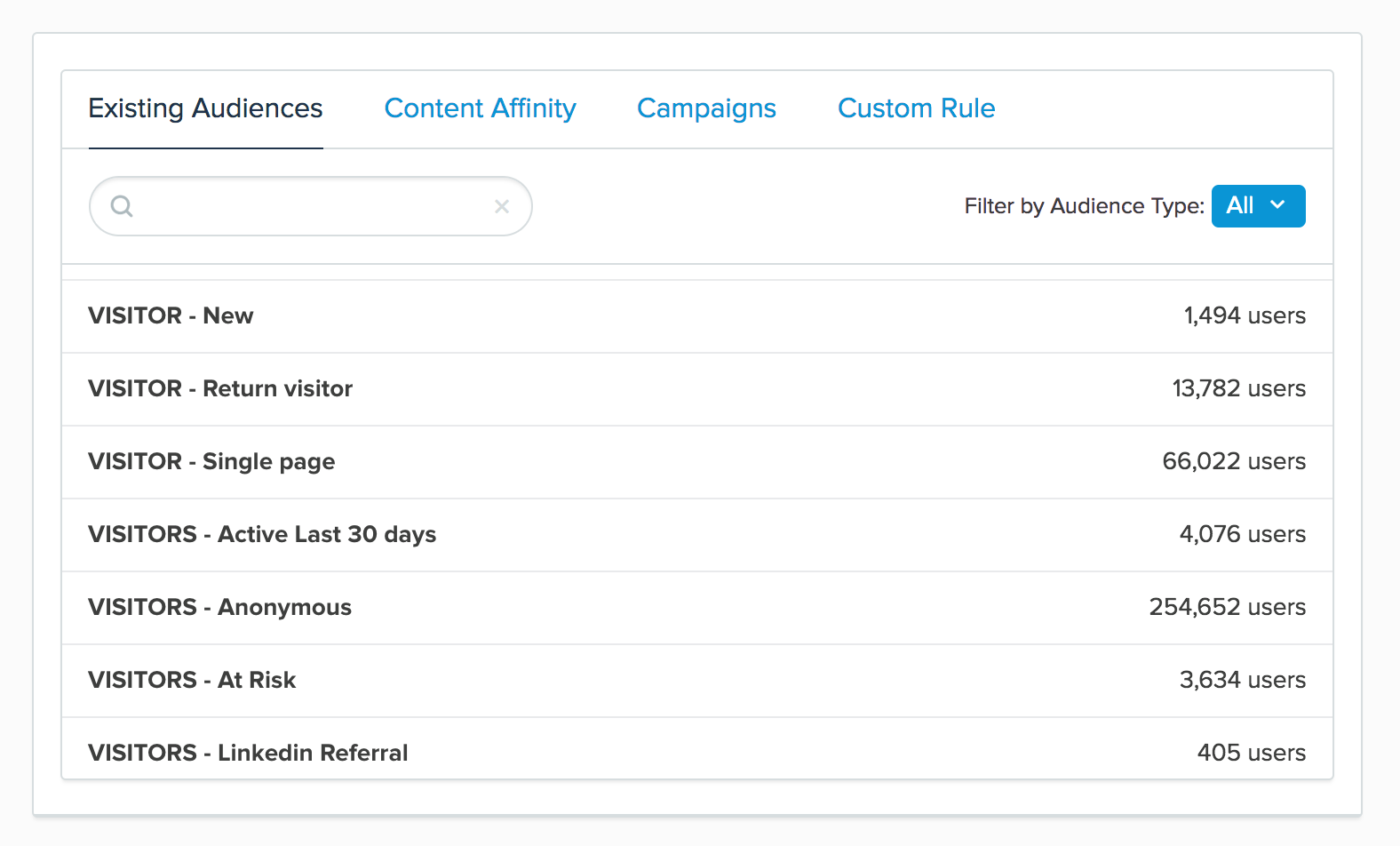This image is a detailed screenshot of the 'Existing Audience' tab on a digital analytics platform. The clean interface features a white background with four primary navigation tabs at the top: 'Existing Audience' (highlighted in white), 'Content Affinity,' 'Campaigns,' and 'Custom Rule' (all in blue). Below these tabs, there's a search bar equipped with a magnifying glass icon on the left and an 'X' icon on the right. To the right of the search bar, it states 'Filter by Audience Type,' accompanied by a blue button labeled 'All' with a downward-pointing arrow indicating a drop-down menu for additional filter options.

The main content area presents seven audience categories with corresponding user counts. The categories are as follows:
1. 'Visitor New,' showing 1,494 users.
2. 'Visitor Return Visitor,' showing 13,782 users.
3. 'Visitor Single Page,' showing 66,022 users.
4. 'Visitors Active Last 30 Days,' showing 4,076 users.
5. 'Visitors Anonymous,' showing 254,652 users.
6. 'Visitors At Risk,' showing 3,634 users.
7. 'Visitors LinkedIn Referral,' showing 405 users.

Each category provides a snapshot of the audience segmentation on the platform, aiding in comprehensive user analysis.